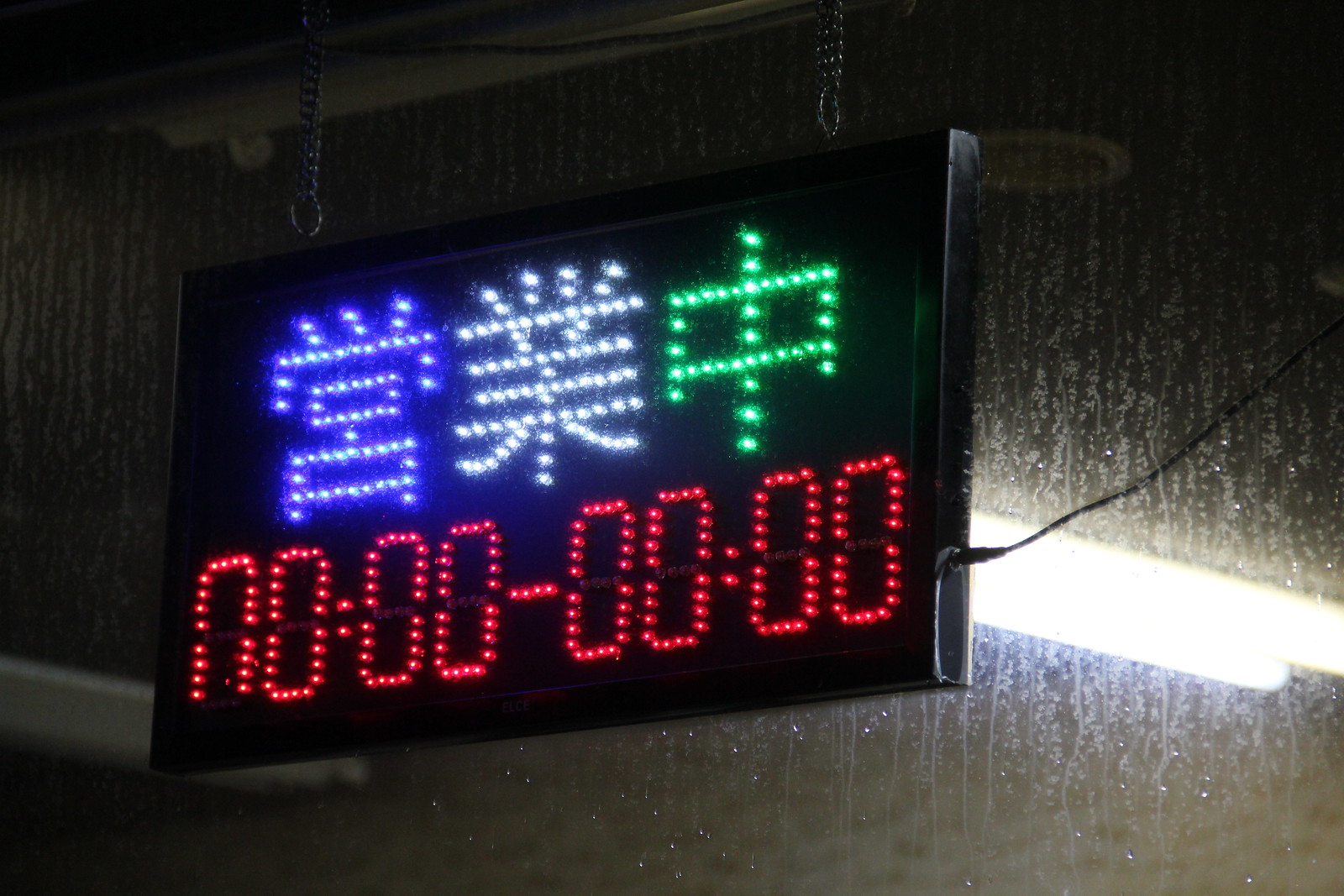A digital sign, possibly in an industrial-looking building or parking garage, hangs from the ceiling by silver chains. The sign, black with LED displays, features three characters at the top—one in pale blue, another in white, and the last in green, which appear to be Asian kanji, possibly Japanese or Mandarin. Below the characters, a row of numbers reads 00:00-00:00 in red, though the bottom part of the first zero is missing. Behind the sign, a window with rainfall visible suggests it is nighttime, with an external light illuminating the scene. The image is dark and somewhat blurry, adding to the damp atmosphere, and a power cord extends from the side of the sign.